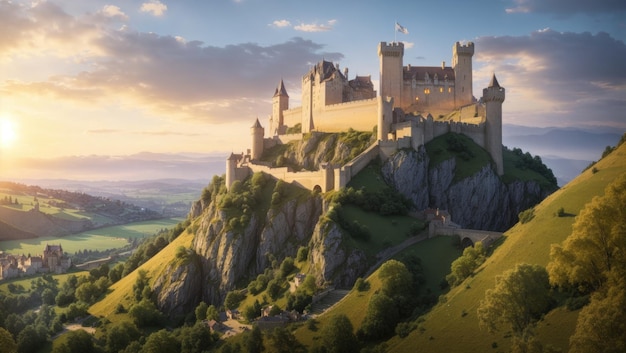This computer-generated illustration features an imposing castle perched atop a steep hill or cliff made of white stone with darker gray accents on its upper sections. The fortress is surrounded by numerous stone towers and spires, and a flag can be seen on one of the central towers. The scene is set during the daytime with the sun low on the horizon, casting a warm light and merging with a partly clear blue sky directly above the castle. Dark gray clouds are visible to the left and right in the far distance. 

At the base of the hill, toward the left, lies a small village with stone buildings, while further down and to the bottom center of the image, there is an even smaller settlement with modest houses. On the center-right side of the image, a stone wall runs through a valley just below the castle. The sheer cliffs beneath the castle reveal the stone beneath but are largely covered in green grass and trees. The foreground reveals a grassy slope, adding depth and texture to the overall scene.